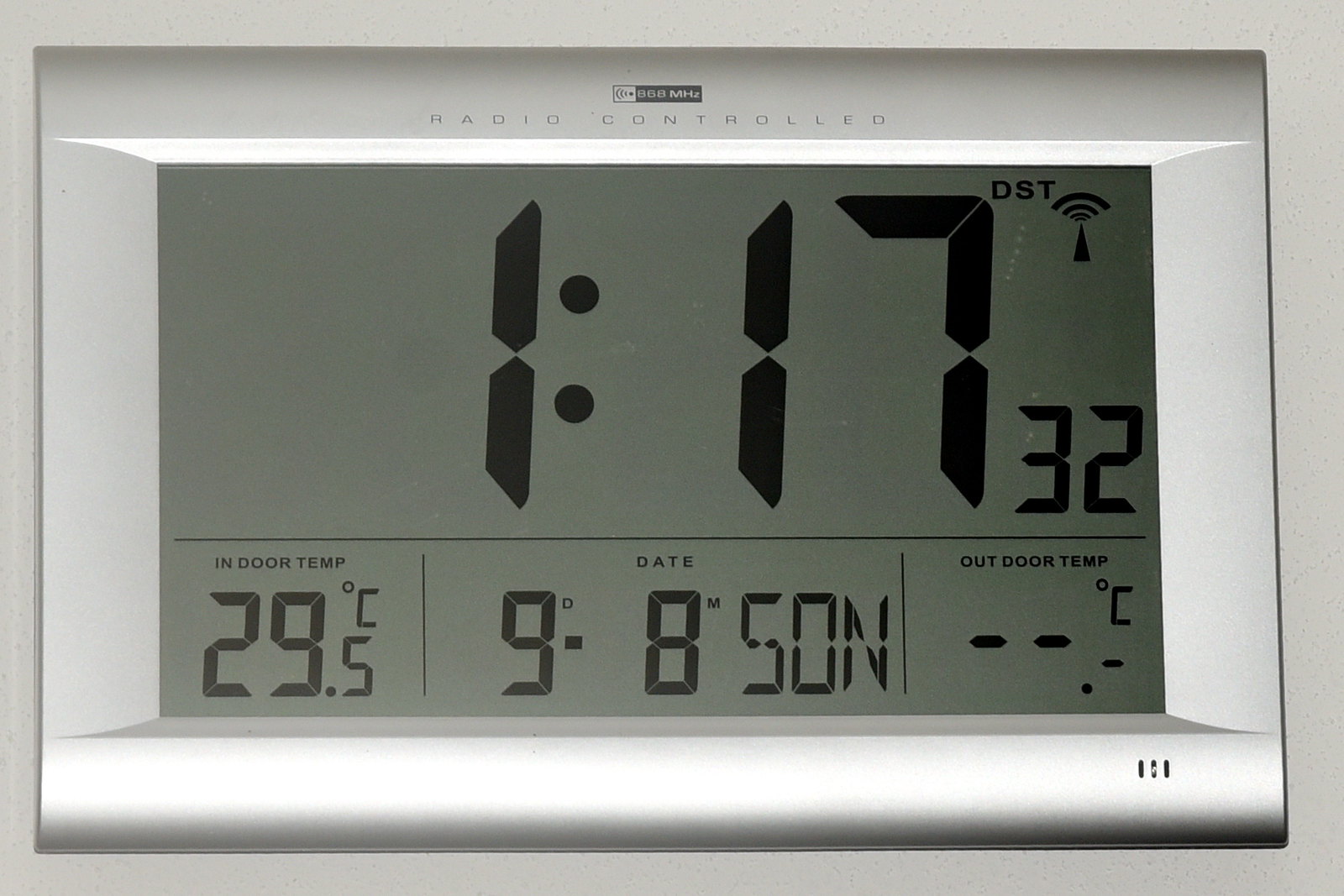This photograph captures a digital display mounted on a wall, framed by a sleek, silver-effect plastic housing. The surrounding area appears pale grey, possibly due to poor lighting. At the top of the display is a logo that is too small to be deciphered, followed by the words "MAGIC CONTROLLED" in neat, capital letters. The digital screen itself features a grey background with black text.

The upper two-thirds of the screen prominently display the time, reading "1:17:32," with the hours and minutes in large digits and the seconds in smaller digits. Adjacent to the '7' and above the '32' second indicator, the letters "DST" and a wireless signal icon are visible.

A thin horizontal line separates this section from the lower third of the display. In the bottom left corner, the indoor temperature is shown as "29.5 degrees Celsius." Moving right, a vertical line divides this segment, leading to the date display, which reads "DATE 9-8" followed by "SON," indicating it is Sunday or "Zondag" in South Africa. Another vertical line marks the next section showing "OUTDOOR TEMP" with placeholders "-- degrees C," suggesting that the outdoor temperature is not currently available.

Finally, in the bottom right corner of the display frame, there are three small holes, likely indicating the presence of a speaker function.